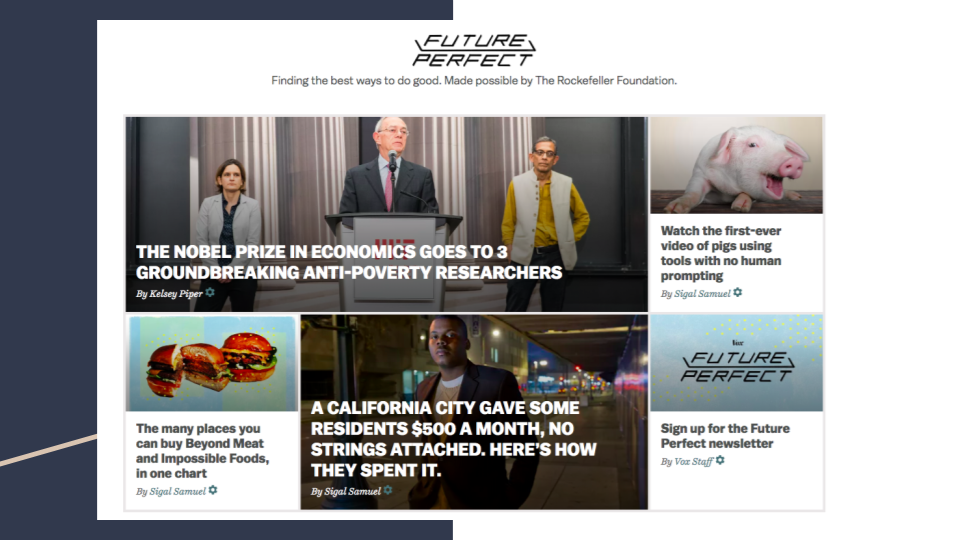This image, sourced from a website, displays an array of articles available for reading. Dominating the layout is a central white rectangle overlaying a dark gray background. At the top, bold text announces "Future Perfect," followed by the tagline "Finding the best ways to do good" and a note that the content is supported by the Rockefeller Foundation. 

On the left side of the image, there is a photograph featuring a speaker at a podium. The speaker, a gray-haired man in a suit coat, is flanked by a woman on his left and another individual on his right. The caption for this image reads, "The Nobel Prize in economics goes to three groundbreaking anti-poverty researchers," authored by Kelsey Piper. 

To the right of this, another notable image features a pig, accompanied by the intriguing headline, "Watch the first ever video of pigs using tools with no human prompting." 

Below these primary stories, there are an additional three articles available for browsing, enriching the variety of engaging content on the page.